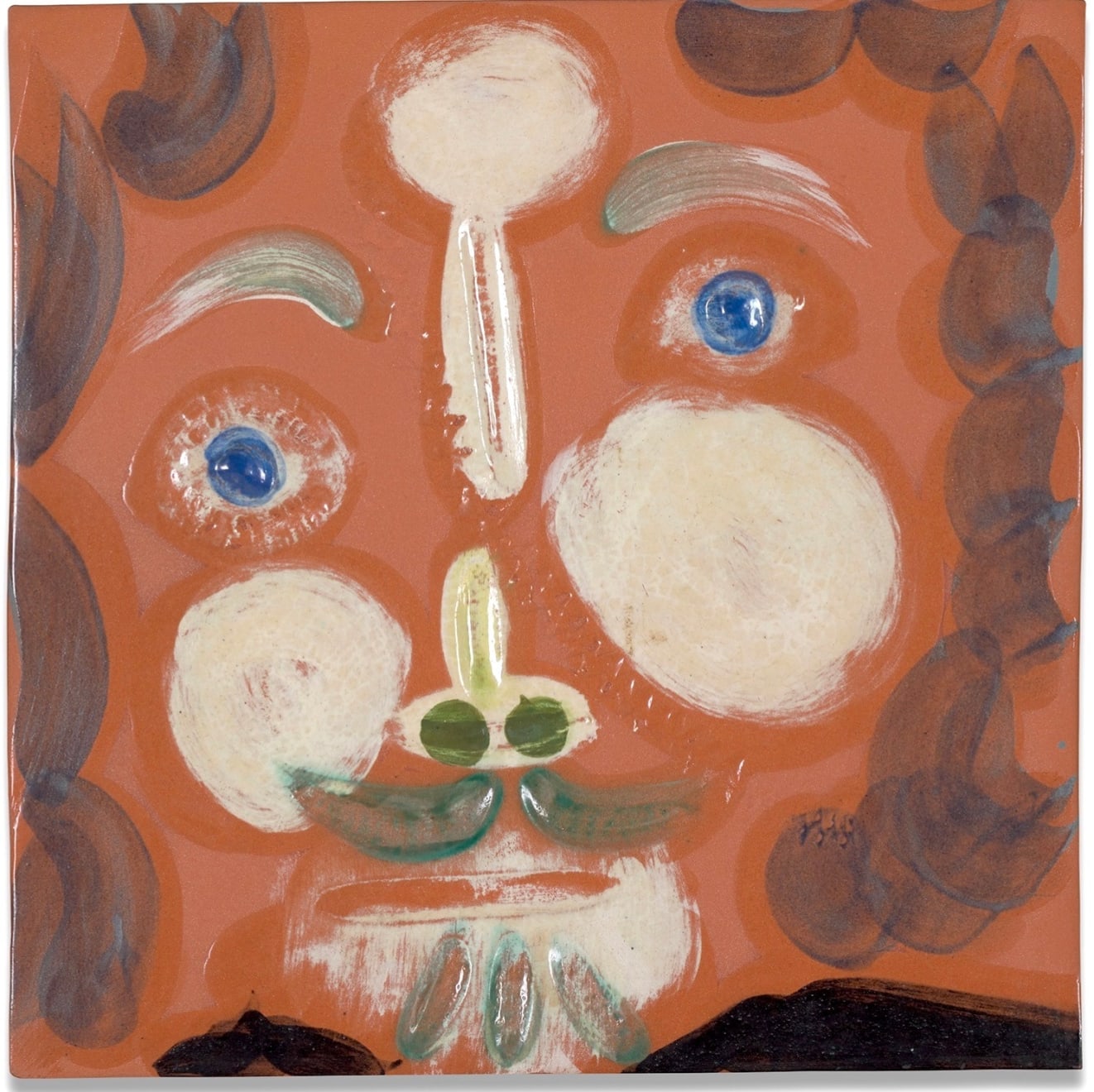This intricate handmade painting portrays an abstract, close-up face rendered on what appears to be orange construction paper, enhanced with a glossy finish. The face, painted predominantly in peach and terracotta hues, exhibits asymmetry, with one side positioned lower than the other. Dark, bluish-gray strokes outline the face, providing depth and complexity. The eyes, irregularly painted in faint white with streaky blue irises, are framed by thin, white eyebrows. The cheeks feature prominently white, asymmetrical circles, the right one significantly larger. Below a small, double-oval nose with green or black nostrils, a green mustache and corresponding greenish-gray beard lines accentuate the lower face. The presence of reflective light over various elements, including a noticeable bubble-like reflection over the nose, adds a textured, almost mixed-media effect. The figure is topped with a mane of similarly colored hair, and one can discern a black shoulder underneath, grounding the portrait in an intriguing meld of abstract and detailed artistry.